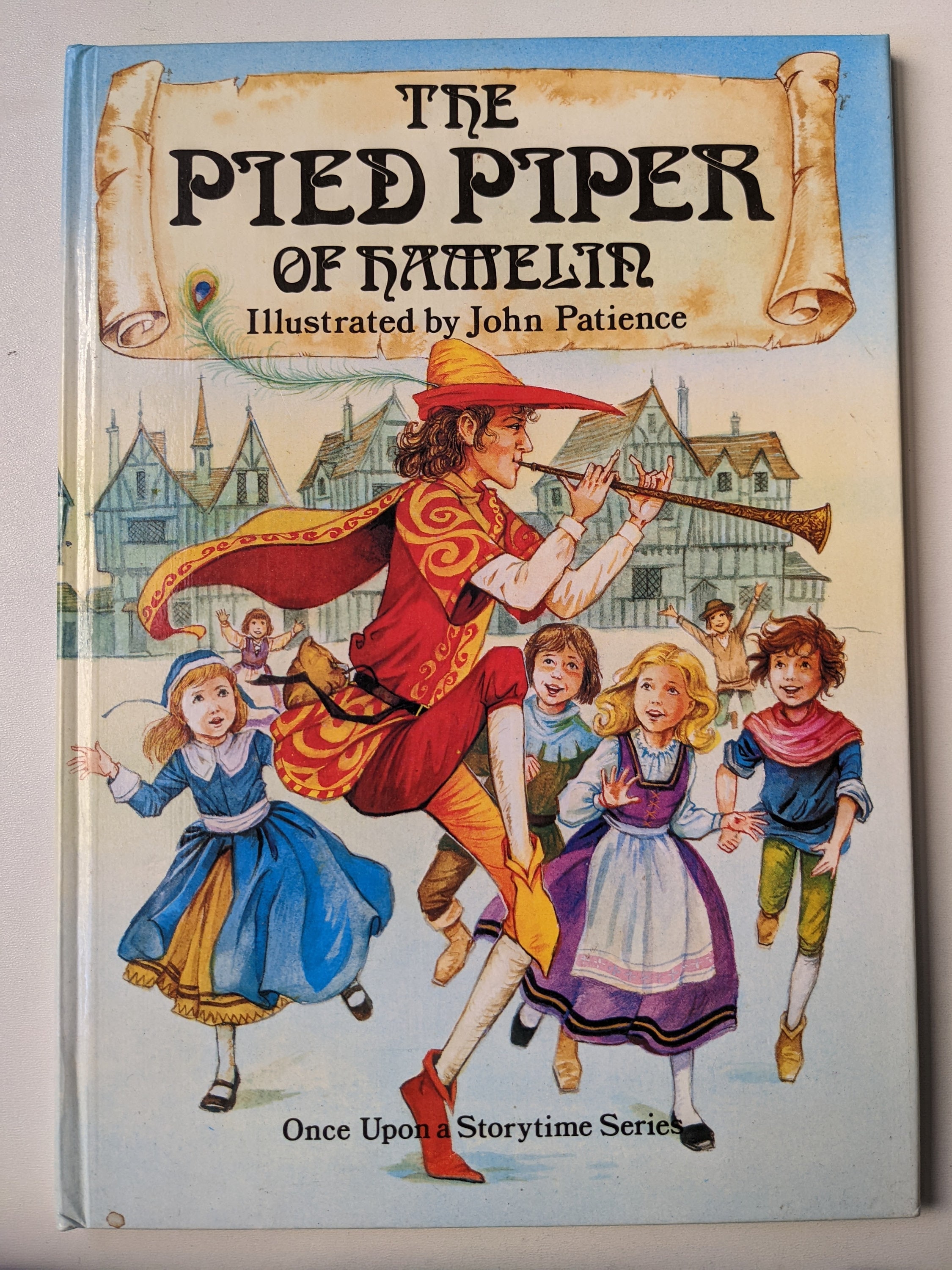The cover of the children’s book titled *The Pied Piper of Hamelin*, illustrated by John Patience, features a detailed and enchanting scene. The main character, the Pied Piper, is a slender man with shoulder-length brown curly hair. He is captured mid-dance, one leg lifted high, as he plays a horn for a group of six enthralled children. The Pied Piper is dressed in vibrant clothing consisting of a pointed orange sombrero and cape, an orange shirt, orange pants, and orange shoes, all accented with golden swirls and curlicues. Surrounding him, the children watch with eager smiles; among them, a girl in a blue dress, a girl in a purple dress, and three boys. The backdrop of the cover depicts idyllic European houses with stucco and peaked roofs, evoking a quaint, Germanic village. The title is prominently displayed in a bold black font, set against a tan unrolled scroll, and at the bottom, the text reads "Once Upon a Storytime Series." The entire scene is richly illustrative, bringing to life the classic tale within.